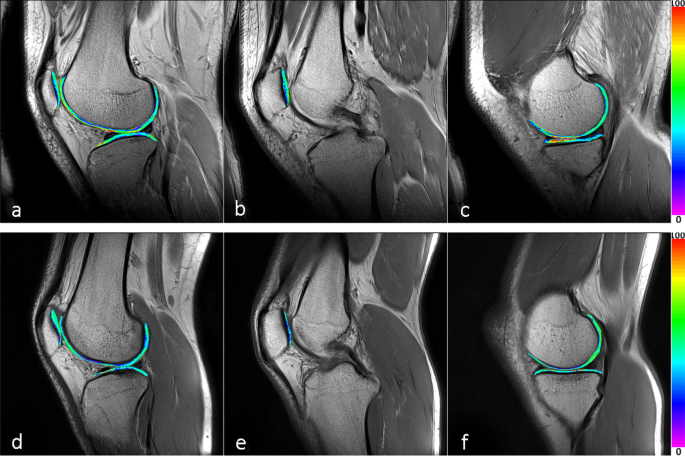This composite image features six detailed scans of knees, labeled A through F, arranged in two rows of three. Each scan reveals a black-and-white imaging style, likely an MRI or PET scan, with highlighted areas in a vivid rainbow spectrum indicating varying intensities. The scans appear to focus on different angles or perspectives of the knees, possibly from different individuals. A color scale is presented alongside images C and F, ranging from purple at 0 to red at 100, depicting intensity levels.

In image A, a largely gray knee structure is overlaid with a striking rainbow line highlighting the cartilage, showing predominant green hues with traces of red and blue around the bones. Image B features a limited rainbow line, localized to the left side, primarily showcasing bluish-green highlights. Image C displays a pronounced rainbow U-shape in the center depicting the cartilage, with a mix of green, blue, and red lines. Image D mirrors the complex rainbow pattern of A, with a central U-shaped highlight leading to a circular line from the bottom, but with less red. Image E offers minimal rainbow coloring, showing primarily the gray structure of the leg with a small sliver of the rainbow line on the left. Finally, image F provides a frontal view of the knee, exhibiting a circular rainbow line around the kneecap, meeting a straight rainbow line from below.

This array of scans provides a multi-faceted view of knee structures, with the rainbow highlights likely indicating different tissue densities or metabolic activities, intensified in images A, C, D, and F. The color gauge emphasizes how the hues correspond to different intensity levels, lending a clear, visual representation of the areas under study.